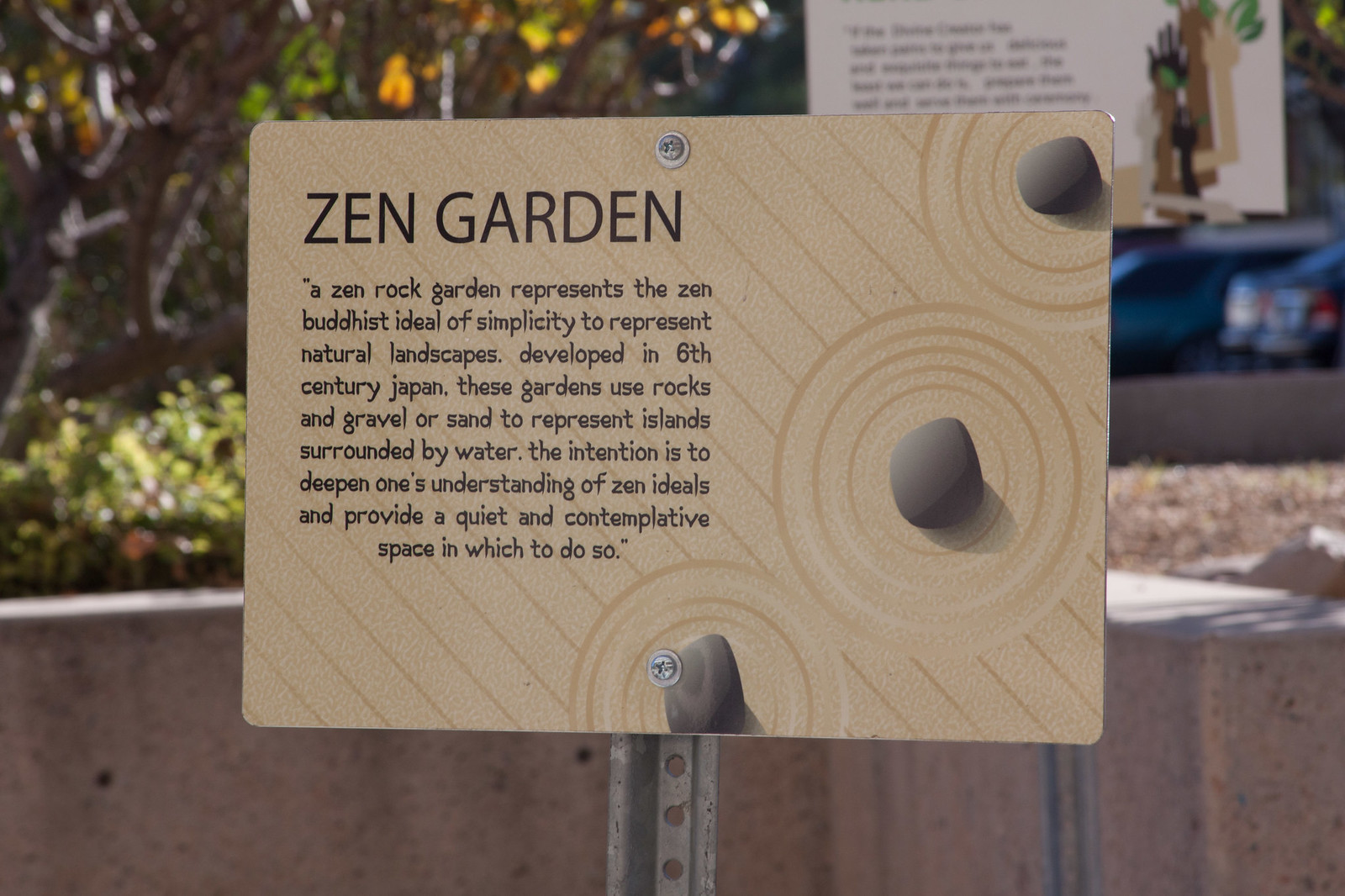The image depicts a scene one might encounter in a botanical garden or a zoological park, featuring an informational sign mounted on a metal signpost. The sign itself is sand-colored, portraying a Zen garden with a graphic illustration of a traditional Zen rock garden complete with rake patterns in the sand. On the right side of the graphic, three rocks are depicted with circular sand patterns, suggesting islands surrounded by water.

Prominently displayed on the top left of the sign, in large black text, are the words "Zen Garden." Beneath this, smaller text provides a detailed description: "A Zen rock garden represents a Zen Buddhist ideal of simplicity, developed in 6th century Japan, to represent natural landscapes. These gardens use rocks and gravel or sand to symbolize islands surrounded by water. The intention is to deepen one's understanding of Zen ideals and provide a quiet and contemplative space in which to do so."

In the background, the outdoor setting hints at a parking lot visible to the right, enhancing the sense that this informational display is part of a larger, potentially serene natural or educational setting.